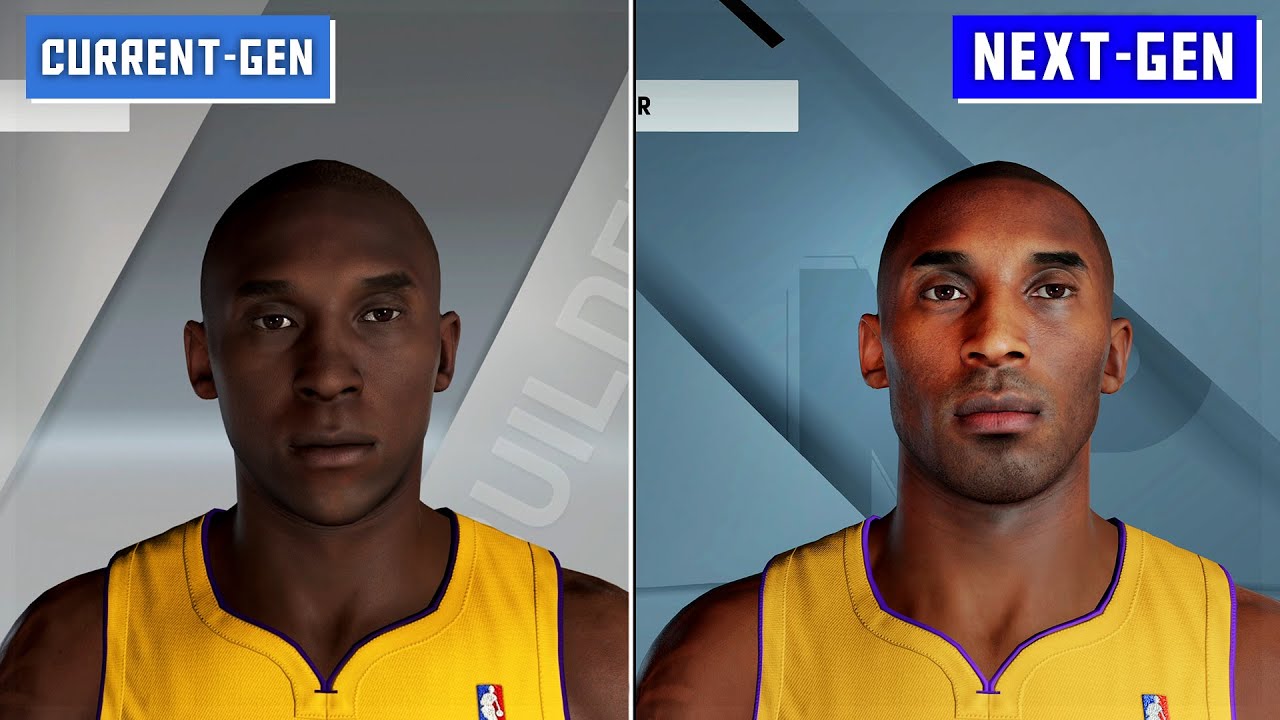This image features two side-by-side photos of a famous basketball player, showcasing a contrast between what is labeled as "Current Gen" on the left and "Next Gen" on the right. In the "Current Gen" photo, the player has a very dark complexion and is wearing his basketball jersey, which prominently displays the NBA logo — red, white, and blue — on the left side. He has a serious expression, staring directly into the camera. Behind him, there is a light-colored sign that appears to read "UILD" and another indistinct light-colored image. The words "Current Gen" are enclosed in a blue box near the bottom of this photo.

In the "Next Gen" photo on the right, the same player is shown with a much lighter complexion, attributed to more light shining on him. His facial features appear slightly more rounded, and his face is evenly illuminated. His head is tilted up a bit more compared to the "Current Gen" image. In the background, there are also diagonal light-colored images, one of which could be interpreted as containing the letters "N" or "M." This side of the image is labeled "Next Gen" in a blue box, mirroring the style of the label on the left. This visual comparison highlights the advancements in lighting or image processing used in displaying the player.